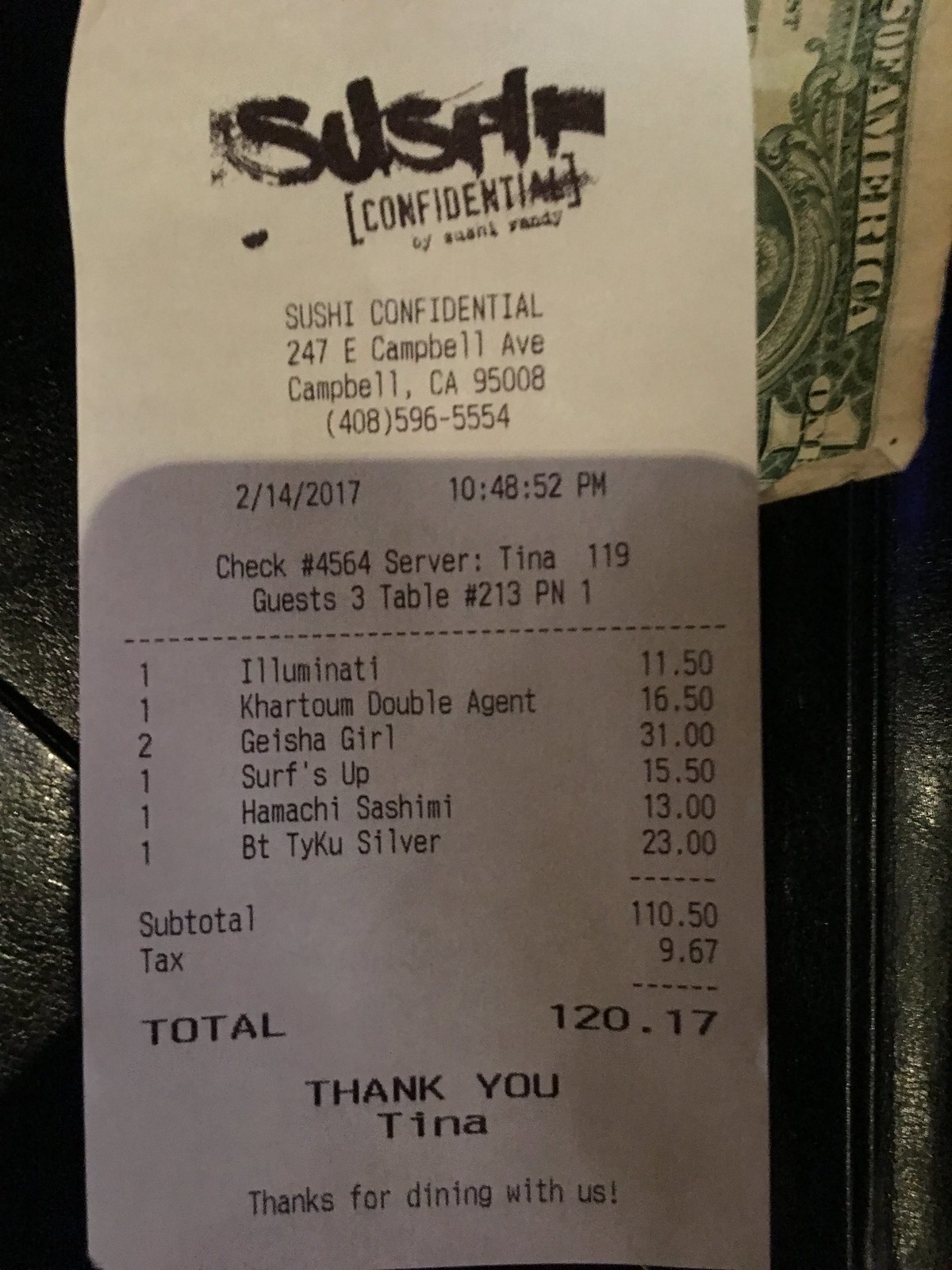The image features a centrally positioned restaurant receipt from "Sushi Confidential" located in Campbell, California, dated February 14, 2017. The receipt, printed in black text on a white background, details the items ordered: Illuminati Cardam, Double Agent Geisha Girl, Surf's Up, and Hamachi Sashimi. The subtotal, tax, and total amount are clearly listed. The background appears to be a leather surface, adding texture to the scene. Behind the receipt, a dollar bill is partially visible, suggesting a tip. The primary colors in the image are black, white, green, tan, and gray, contributing to the realistic portrayal of a typical dining payment scenario.